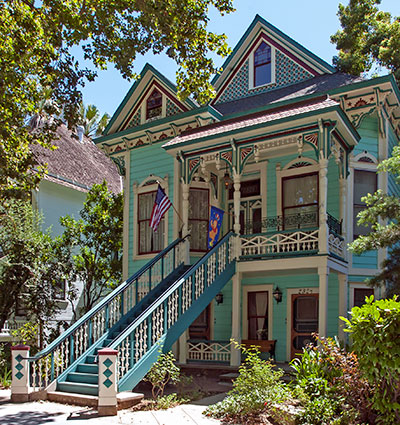This photograph captures a picturesque, ornate mansion with an intricate design reminiscent of a bygone era. The light blue, almost aqua-colored exterior of the two or three-story house is framed by trees on both sides. A long, elegant staircase, adorned with blue railings, ascends to the second-floor main entrance. On either side of the stairs, there is an American flag and a blue flag with a yellow and red logo. The house features a pointed roof with windows, adding to its majestic appearance. The foreground includes some shrubs, and the entire scene is set against a clear sky, bathed in bright daylight. The image exudes a timeless charm and showcases the intricate architectural details beautifully.